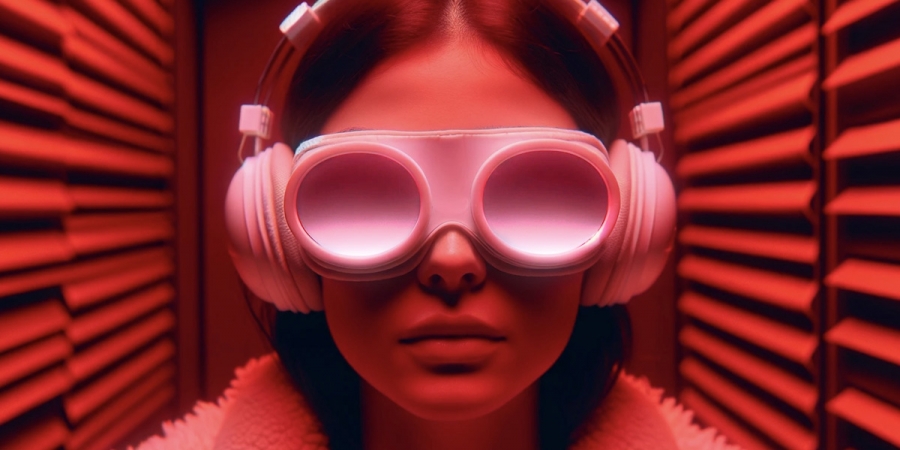This image portrays a young girl, possibly a teenager, set against a highly stylized red backdrop that bathes the entire scene in a reddish hue. The ambient light makes it challenging to discern exact colors but leaves a striking monochromatic impression. The girl, with dark, possibly brown or even red hair, has it parted in the middle. Her profile is captured with her mouth closed, looking towards the camera.

She dons a pair of large, opaque, solid pink goggles, reminiscent of those used for welding, obscuring her eyes completely. Over her ears sit a pair of pink closed-back headphones, connected by a headband running over her head. The headphones' design brings to mind shapes like half donuts or bagels.

Completing her attire, she wears a jacket that appears to be made of a fluffy, textured fabric, likely Sherpa, with a Sherpa pile-style finish. The exact color of the jacket is ambiguous due to the red lighting, but it could be pale or white in a neutral setting.

The background features ribbed or shutter-like structures on either side, possibly resembling soundproofing panels or abstract washboard patterns, enhancing the image’s futuristic and surreal ambiance. A door or wall, also masked in red light, sits behind her, adding to the scene's overall enigmatic and dreamlike quality.